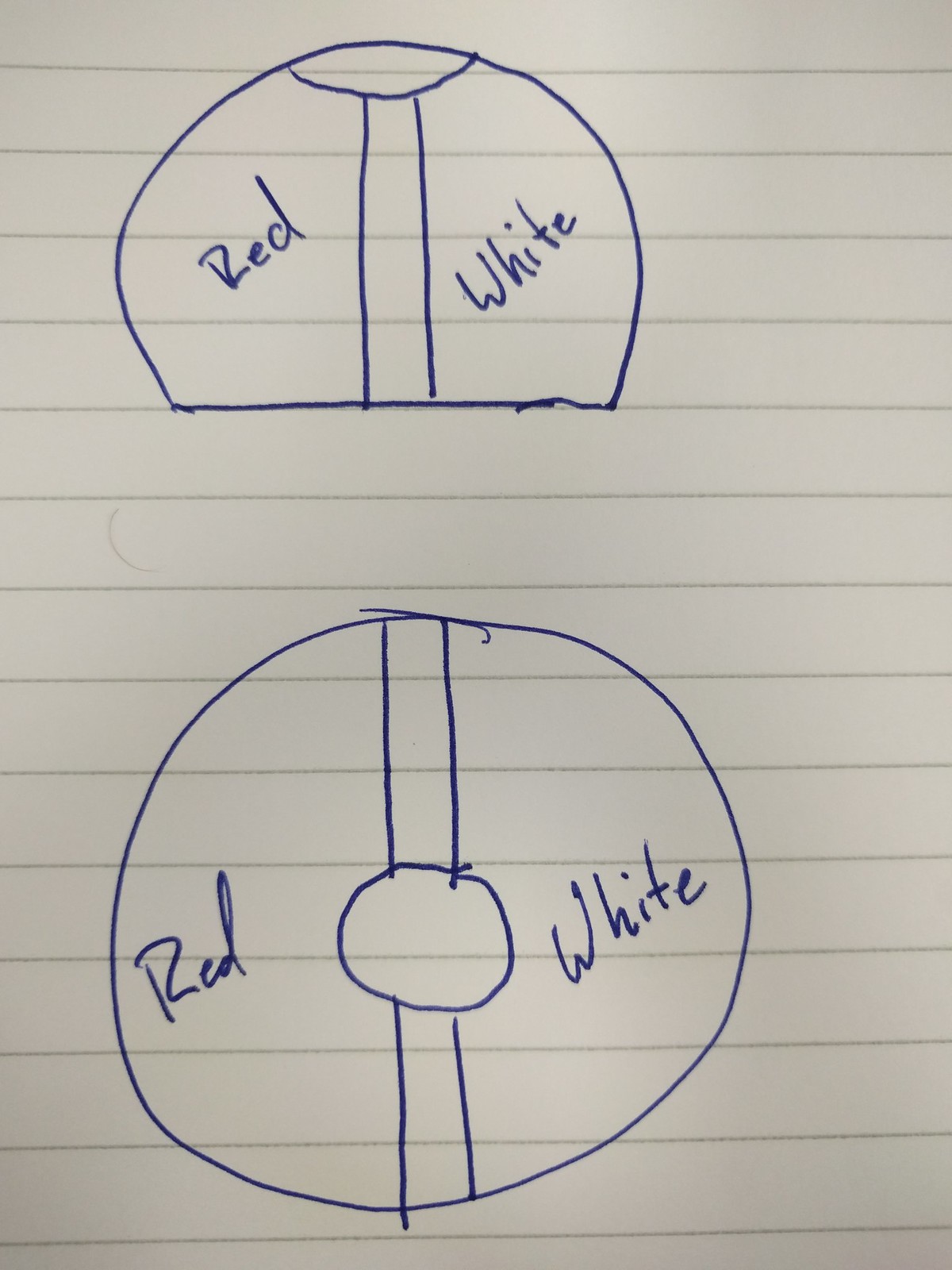A piece of lined notebook paper features a detailed blue ink sketch at the top, presenting two perspectives of the same object. The first drawing, viewed from the side, resembles an incomplete sphere with the bottom third removed. Two lines bisect the center, converging into an arc that curves downward, suggesting a three-dimensional form. The left segment of this sketch is labeled "red," while the opposite segment is labeled "white."

The second drawing, oriented directly below the first, offers a top-down view of the same object. Here, the circular outline and intersecting lines are seen from above, maintaining the same "red" and "white" designations as before. Notably, cursive is used for the word "red" in this view, but "white" is consistently written in standard print in both illustrations. The paper itself has a subdued, dim appearance, and the sketches appear preparatory, hinting at a future project.